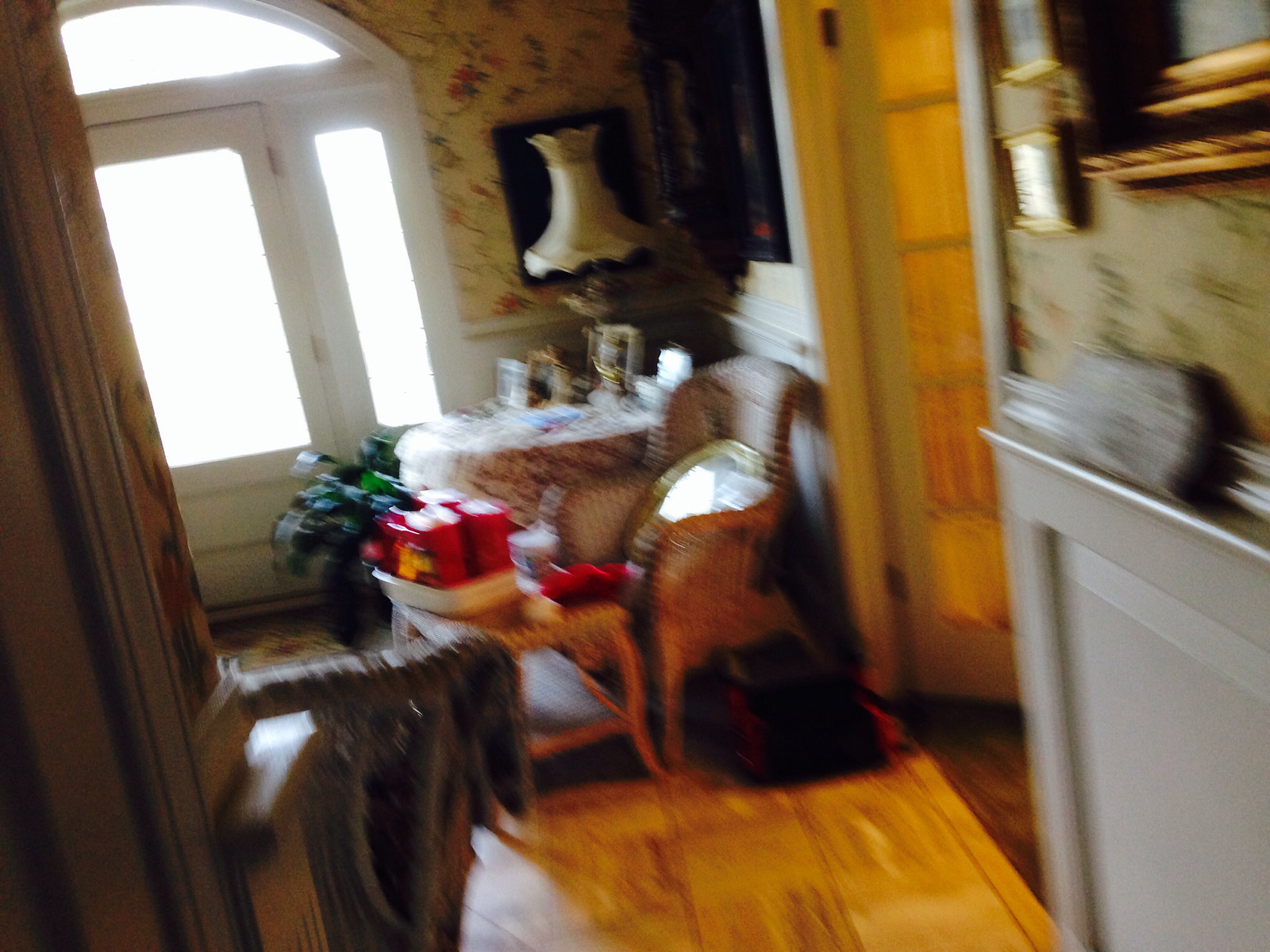In this slightly blurry and fuzzy indoor image, the central focus is a chair with a round mirror placed on its seat. To the left of the chair, there is a leg stool with indistinct items on its surface due to the low quality of the image. Behind the chair, a round table is visible, also holding various unclear items, with a discernible lamp positioned on it. Despite the blurriness, the primary objects in the room are identifiable.